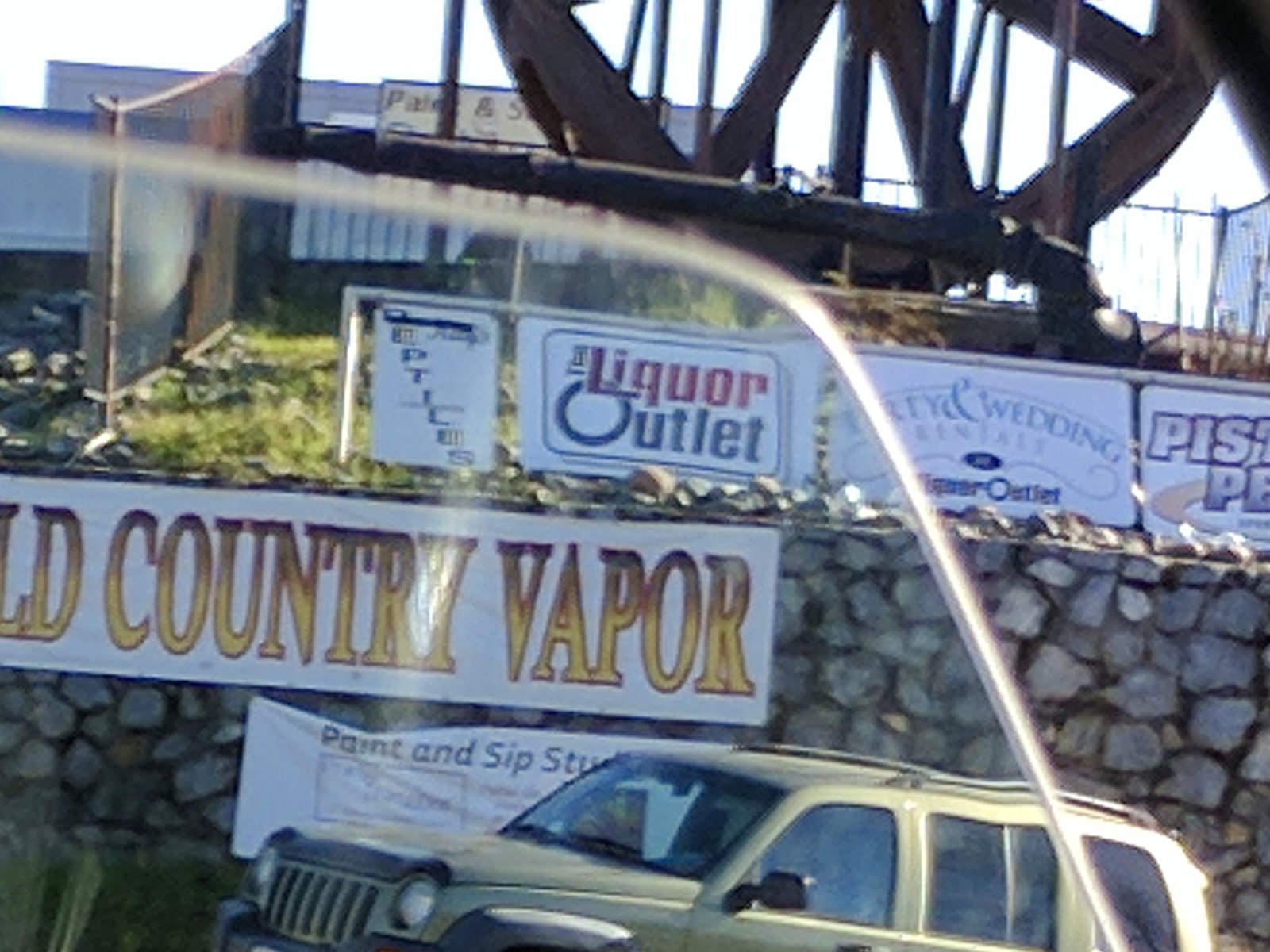This outdoor color photograph captures the scene from the bottom up. At the very bottom, there is a gray-colored car, possibly a station wagon, where only the hood and roof are visible. Directly behind the car stands a stone wall with a large sign that reads "Old Country Vapor" in gold letters set against a white background. Above this main sign, several smaller signs are posted, one of which reads "The Liquor Outlet," while the text on the other three signs is too small to discern. In the background, a hill rises above the wall, and further up, part of what seems to be a bridge is visible. The sky overhead is a muted gray, lending a subdued tone to the scene.